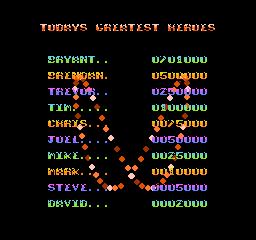The image is a winner's screen from a computer game displayed after completing a round. The background of the screen is black, providing a stark contrast that highlights the text and graphics. At the top of the screen, the title "Today's Greatest Heroes" is prominently displayed in bold red letters. Below the title, a list of the top ten players is neatly arranged.

The list is on the left side of the screen, with each player's name and corresponding score beside it. In striking green, "Bryant" is at the top with an impressive score of 701,000 points. Beneath him, "Brendan" is displayed in orange with a score of 500,000 points. Following them is "Trevor" in purple, who has achieved a score in the range of 200,000 points. The remainder of the list includes other players, each name and score alternating between green, purple, and orange colors.

Adding an element of excitement, a series of red squares arranged in a swirly pattern decorate the screen, adding a dynamic and engaging visual effect to the otherwise text-heavy display. This artistic touch enhances the celebratory nature of the winner's screen.